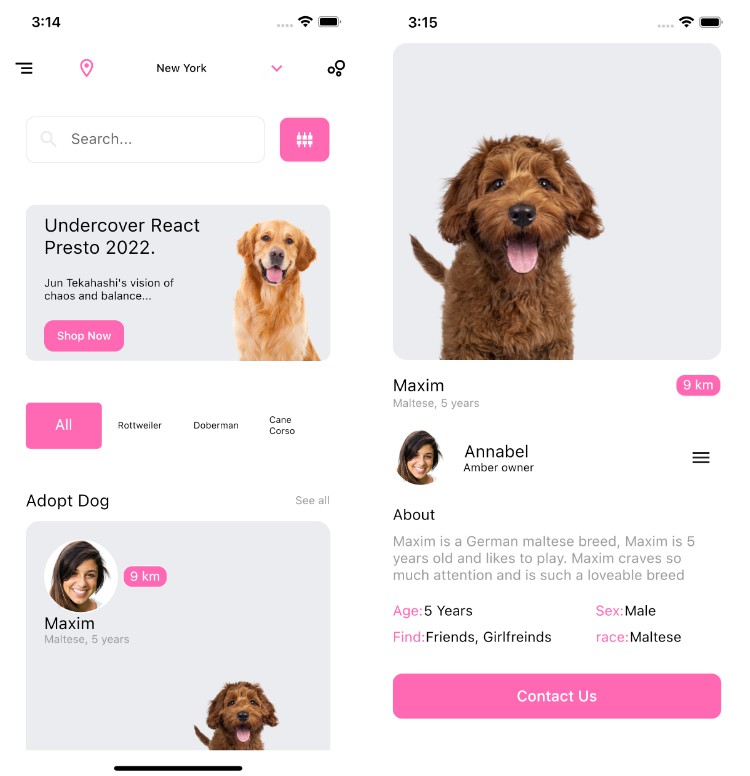This composite image consists of two mobile phone screenshots, side by side, displaying a website dedicated to dogs. The screenshots are nearly identical, differing only by the time shown in the top bar: 3:14 PM on the left and 3:15 PM on the right.

### Left Screenshot Description:
- **Top Bar**: Displays the location "New York" in black font.
- **Search Field**: Located below the top bar, accompanied by a magnifying glass icon on the right, and a pink button on the left featuring symbols resembling spark plugs.
- **Gray Rectangle**: Below the search field, a gray rectangle contains an image of a cute golden retriever.
  - **Text within Gray Rectangle**: 
    - **Upper Left Corner**: "Undercover React Presto 2022, John Takahashi's vision of chaos and balance, shop now" (puzzling call-to-action text).
- **Option Buttons**: Below the gray rectangle are clickable options labeled "All," "Rottweiler," "Doberman," and "Cane Corso," with "All" selected.
- **Section Title**: Below the options, "Adopted dog" appears in black font.
- **View Option**: To the right of the section title, "See all" is in gray font.
- **Gray Square**: Below the section title is a gray square featuring:
  - **Profile Circle**: A circular image of a Latina woman in her twenties with brown hair.
  - **Profile Detail**: Underneath the profile circle, "Maxim" appears in black font, along with the word "Maltese".

### Right Screenshot Description:
The right screenshot mirrors the left, with the following notable differences:
- **Time in Top Bar**: Displays 3:15 PM (one minute later than the left screenshot).

Overall, the composite provides a snapshot of an engaging dog-centric website interface with search and display features, user interaction options, and profile highlights.